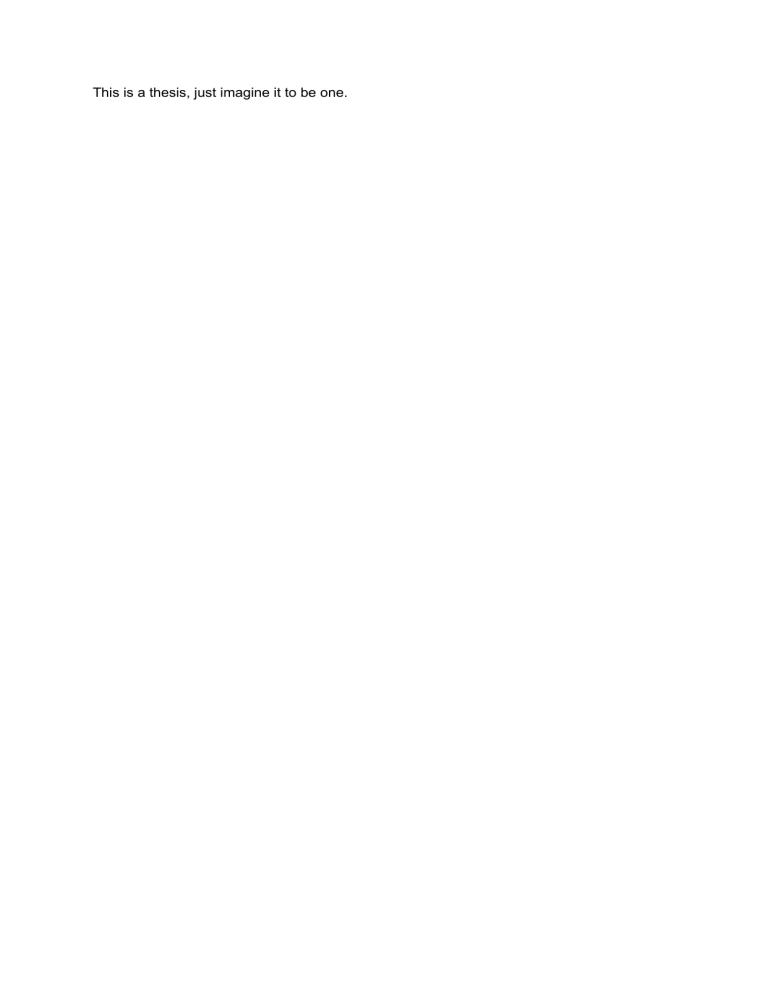The image showcases a minimalist design with a completely white background devoid of any borders. Positioned towards the upper portion of the frame is a single line of small text that succinctly reads, "This is a thesis, just imagine it to be one." The placement of the text leaves a substantial expanse of empty white space below, amplifying the simplicity and sparseness of the overall composition. The stark contrast between the minimalistic text and the vast white space invites contemplation and curiosity about the deeper meaning behind the statement.